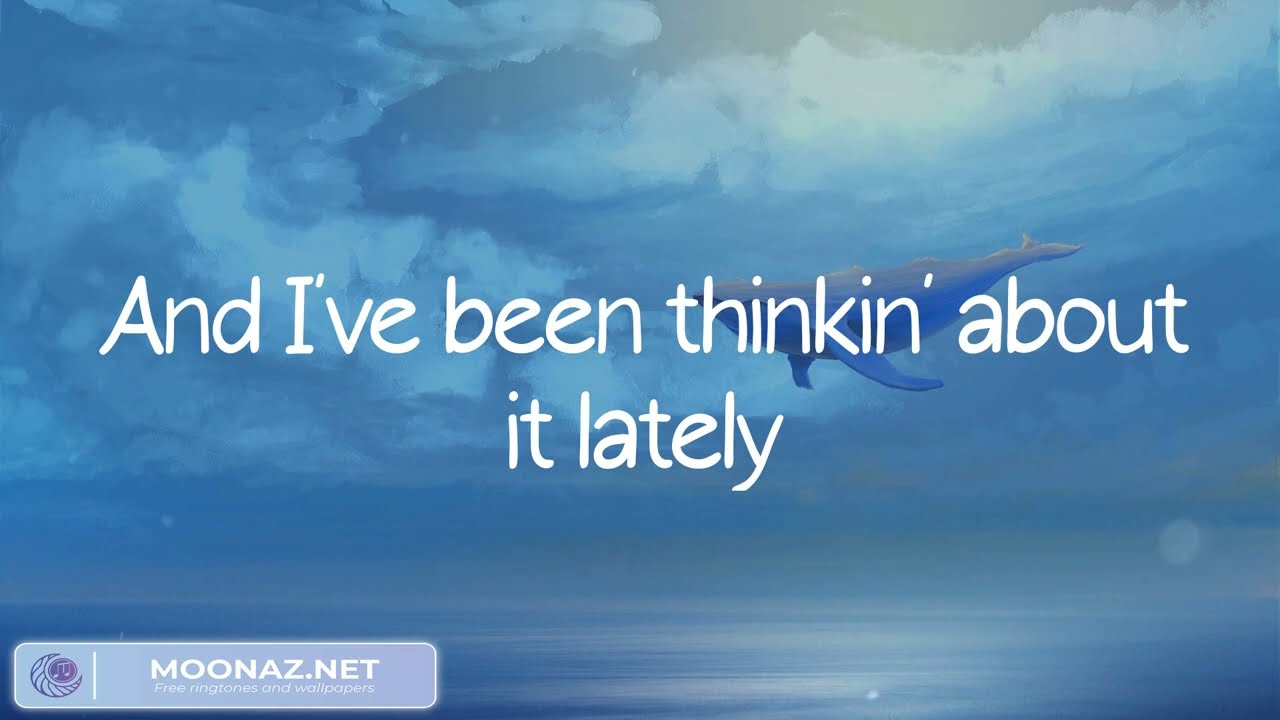The image is a predominantly blue-themed artwork that merges elements of sky and ocean in a surreal, dream-like composition. At the center of this image, large white text reads, "and I've been thinking about it lately," with the words split across two lines. This text partially obscures a dark blue whale, which appears to be gliding through fluffy blue and whitish-gray clouds. The background features a harmonious mix of dark and light blue tones, with the ocean visible below, blending seamlessly into the sky. At the bottom left corner, there is a watermark enclosed in a rectangular or oval shape that reads "moonaz.net, free ringtones and wallpapers," accompanied by a logo of a crescent moon embracing a circle with a music note inside.